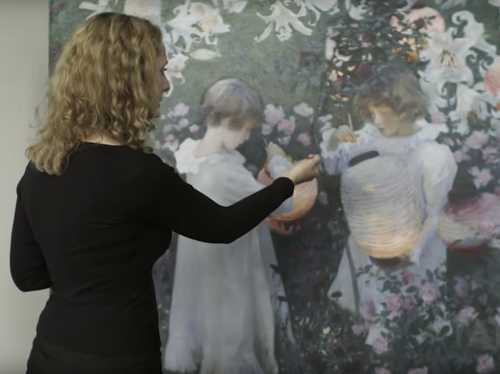In this image, a woman in her late 30s to early 40s, with shoulder-length, curly blonde hair and dressed in a long-sleeved black blouse and black bottoms, stands in front of a large art deco-style painting. She appears to be gesturing or possibly touching up the painting, which depicts two children, one boy and one girl, in long white outfits. The girl is holding a see-through lantern glowing with multiple lights, likely filled with fireflies, while the boy holds a similar lantern-like object, only partially visible due to the woman’s arm. The background of the painting features muted colors resembling a colorized black-and-white photograph, with detailed designs of plants and flowers, giving an impression of a garden scene.